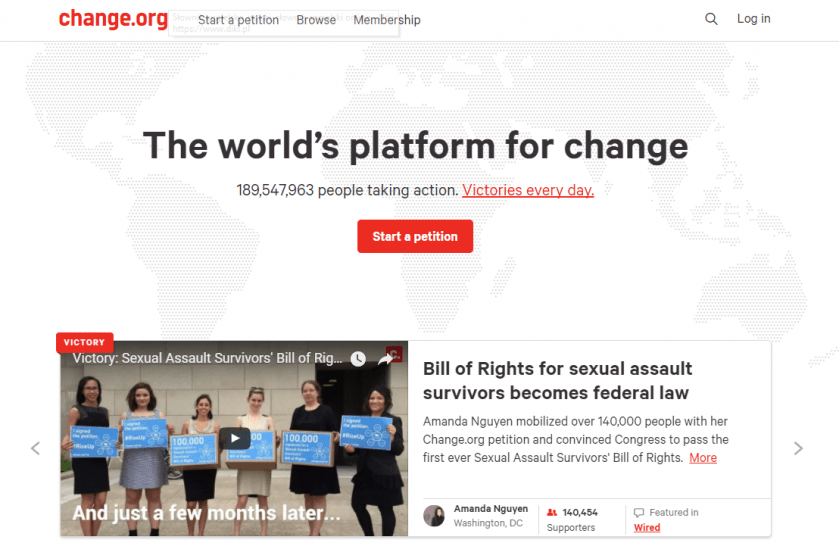This image captures a significant moment in the fight for sexual assault survivors' rights, featured on a webpage dedicated to change. On the lower left side, there is a video thumbnail showing a group of women holding blue signs that read "Victory: Sexual Assault Survivors' Bill of Rights." This video appears to be aimed at informing viewers about the successful passage of the first-ever Sexual Assault Survivors' Bill of Rights, achieved after several months of advocacy and pressure on Congress.

To the right of the video, a bold header states, "Bill of Rights for Sexual Assault Survivors Becomes Federal Law." Below the header, text explains that Amanda Nguyen mobilized over 140,000 individuals through a Change.org petition, successfully convincing Congress to enact this groundbreaking legislation. Below this, an image shows Amanda Nguyen in Washington, D.C., surrounded by supporters. The caption indicates that almost 141,000 people were involved in this effort and that the story was featured in Wired magazine, with a hyperlink provided to the Wired article.

Above this section, large text on a watermarked globe background proclaims, "The World's Platform for Change," highlighting that 189 million people are taking action and experiencing victories daily, with the phrase "victories every day" underlined in red. The webpage also includes a button to start a petition and a login option at the top-right corner. The top-left corner prominently displays the Change.org logo, with additional options to start a petition, browse existing petitions, and explore membership benefits.